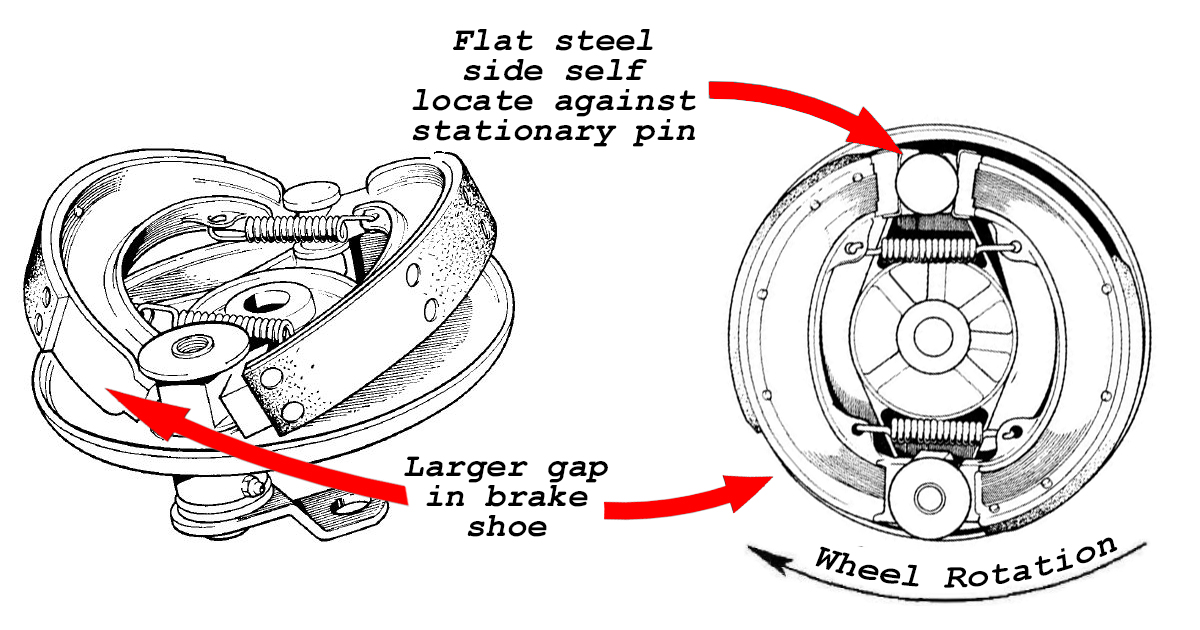The image depicts a detailed illustration of a drum brake system, featuring two distinct views: a 3D isometric perspective and a top-down, plan view. Both illustrations are rendered in black and grey, set against a white background. The 3D view on the left showcases the internal components of the drum brake, including the brake pads, two springs, and a circular pin. The top-down view on the right highlights the arrangement and positioning of these parts.

In the image, text annotations are provided in black, accompanied by red arrows for clarity. The upper annotation reads, "Flat steel side self-locate against stationary pin," with an arrow pointing to a specific component in the top-down view. The lower annotation states, "Larger gap in brake shoe," and directs attention to the corresponding area on the 3D view of the brake. These annotations help explain the function and assembly of the drum brake components. Red is also used to denote arrows that point towards significant parts in each illustration, enhancing comprehension of the brake system's mechanics.